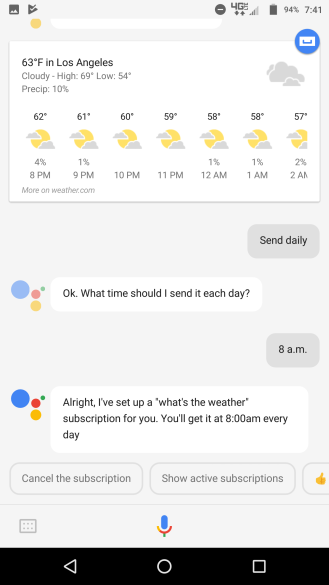Screenshot of a mobile phone in landscape mode featuring multiple elements. On the top of the screen, there's a notification from a video player application, symbolized by a large minus sign inside a circle. The phone displays 4G LTE connectivity with four out of five bars and a battery level of 95%. The time is 7:41 PM.

Below the notification area, there is a weather widget showing the current conditions in Los Angeles: 63°F and cloudy with a high of 69°F and a low of 54°F, and a 10% chance of precipitation. Additionally, there is an hourly forecast from 8 PM to 2 AM, displaying a temperature range from 62°F at 8 PM gradually decreasing to 57°F by 2 AM.

In the messaging app, the user is having a conversation with a contact named "Send Daily." The user asks, "What time should I send each day?" and receives a reply of "8 a.m." Following this, "Send Daily" confirms, "All right, I set up a weather subscription for you. You'll get it at 8 a.m. every day." Below this conversation, there are buttons labeled "Cancel Subscription," "Show Active Subscriptions," and a thumbs-up icon. 

At the bottom of the screen, there is a voice chat option, as well as the standard navigation buttons for back, home, and menu, commonly found on smartphones.